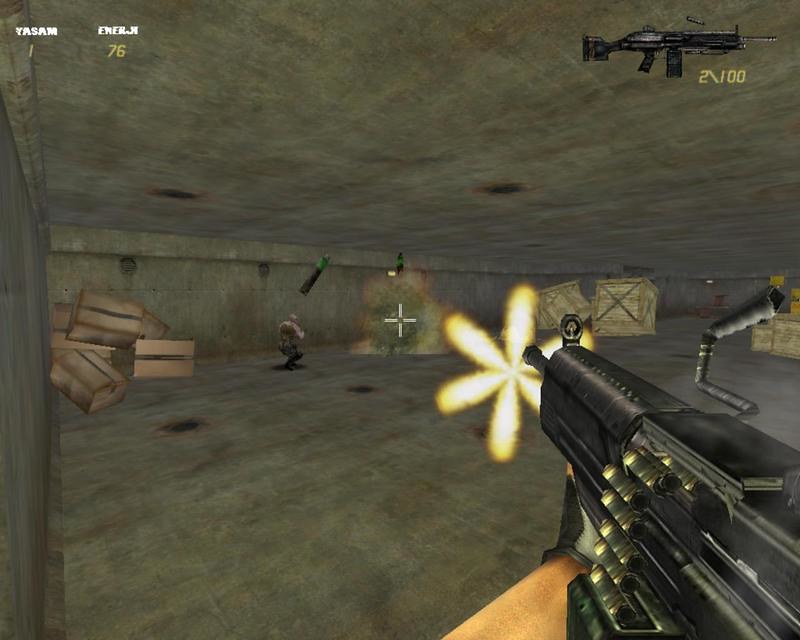A screenshot from an old-school first-person shooter video game showcasing crude, low-resolution graphics. The scene is set in a grey, warehouse-like room cluttered with covered boxes and wooden crates. The player-character, seen from a first-person perspective, wields a machine gun, actively firing at distant enemies. The character's arms are visible, revealing Caucasian skin and black gloves. To the left of the crosshairs in the center of the screen, another adversary, possibly a monster or human, can be seen. In the lower right corner of the screen, a small image of the machine gun is displayed, accompanied by ammunition indicators showing "2 out of 100" rounds remaining.